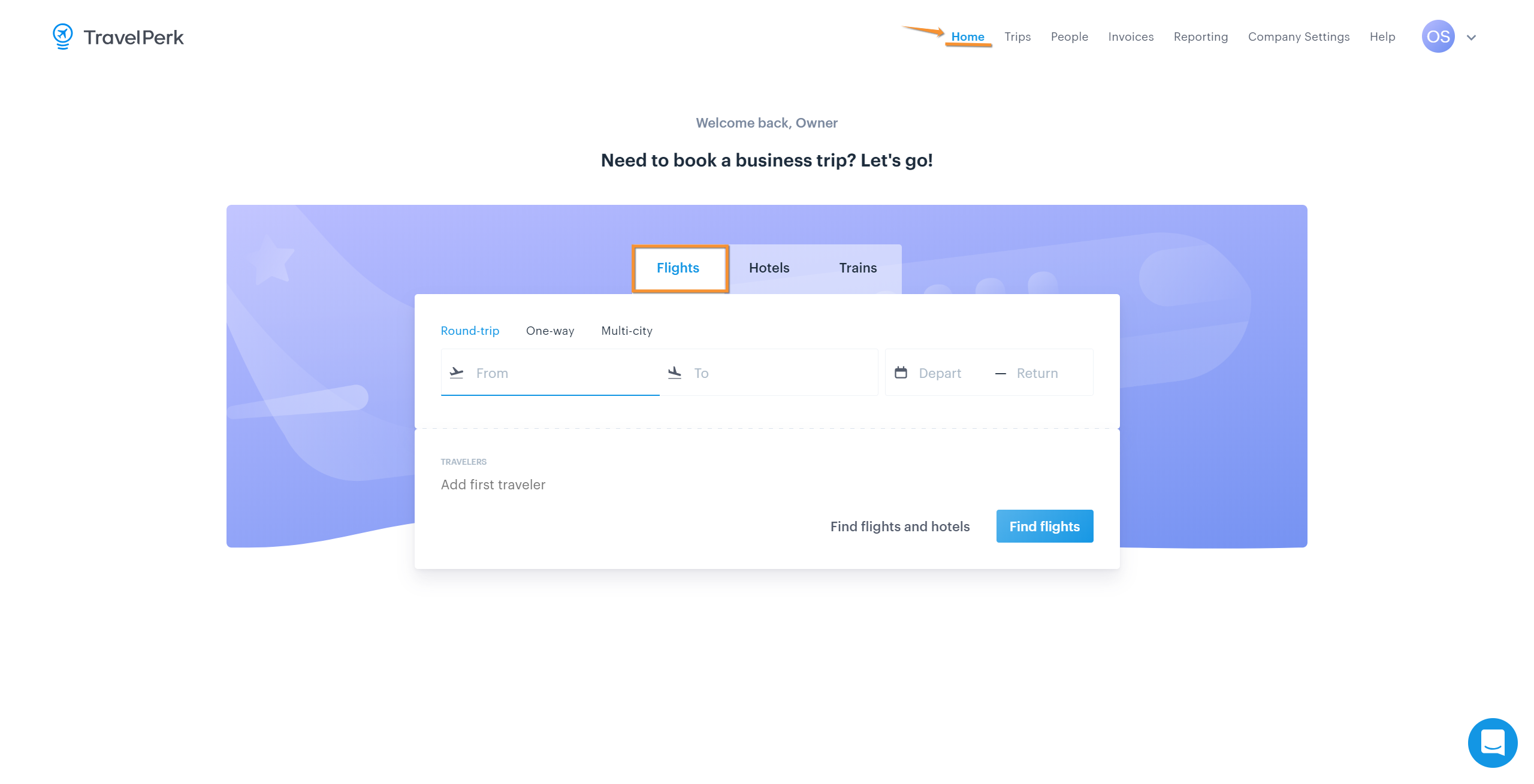In the top left corner of the screen, a circular icon features a plane with two curved lines beneath it, all rendered in blue. Adjacent to the icon is the text "TravelPerk," styled in blue capital letters with capital 'T' and 'P'. Below the logo, a navigation menu is present. An attention-drawing yellow arrow points towards the 'Home' menu item, which is highlighted with a yellow underline. The 'Home' option is prominently displayed in blue, while the other menu items—'Trips,' 'People,' 'Invoices,' 'Reporting,' 'Company Settings,' and 'Help'—are listed sequentially.

To the far right of the menu, an 'OS' icon is visible, characterized by white text inside a purple circle. An adjacent dropdown arrow signals a menu, with the text "Welcome back, Owner" in light gray, followed by "Need to book a business trip? Let’s go!" in bold black text.

Below the navigation bar, a visually appealing rectangle exhibits a watermark design of an airplane against a gradient background shifting from lilac to dark blue periwinkle. The rectangle houses a pop-up box divided into three tabs: 'Flights,' 'Hotels,' and 'Trains,' with the 'Flights' tab currently active, highlighted by a gold border. The 'Flights' section provides multiple options: 'Round-trip,' 'One-way,' and 'Multi-city,' with 'Round-trip' selected and highlighted in blue. Input fields for flight information labeled 'From' and 'To' sit below, marked by a blue line extending from an airplane icon.

Further details include a small calendar icon annotated with 'Depart' and 'Return' headers, accompanied by minus buttons and an option to add travelers starting with 'Add first traveler'. At the bottom of the pop-up, two actionable buttons are displayed: 'Find Flights and Hotels,' and another 'Find Flights' button in blue with white text. Rounding out the interface, a speech bubble icon with a smiley face is situated in a circular icon at the bottom right-hand corner of the screen, signifying a chat feature.